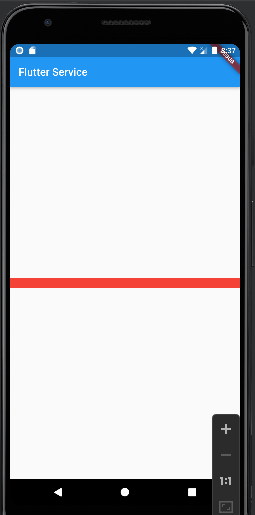The image features a smartphone against a gray background. The phone has a slim black border along the top edge and a slightly thicker gray border down the sides. Just inside the outer border, there's an additional thin black border. At the top left of this black border, there is a small gray square with a blue dot inside it. In the center of the top edge is a speaker slit, approximately an inch wide and gray in color. Beneath the black border is a thin dark blue line.

On the screen, the top left corner displays a white circle and the top right corner has a small white square. The time, shown in white, reads "8:37". Alongside the time are icons: a battery icon indicating full charge, an internet signal icon showing half signal, and a Wi-Fi icon showing full signal. Diagonally descending from the top left to right is a red strip, positioned around the area displaying the time. The strip includes white text that is too small to be legible.

Below this section, there is a light blue area, about an inch thick, with the words "flutter service" on the left side. The red strip slightly overlaps into this blue section. Following this, the lower part of the screen is predominantly white, except for about an inch at the bottom. Across the center of this white area runs a red bar, approximately a quarter of an inch wide. 

The bottom inch of the phone’s design is black. On the left side, there’s a white triangle pointing to the left, a white circle, and a white square. From the right corner running upwards about two inches, then turning to the left for about an inch, and then downwards, there is a dark gray element. This dark gray area features a light gray plus sign at the top, a minus sign in the middle, the notation "1..1", and a small square at the bottom.